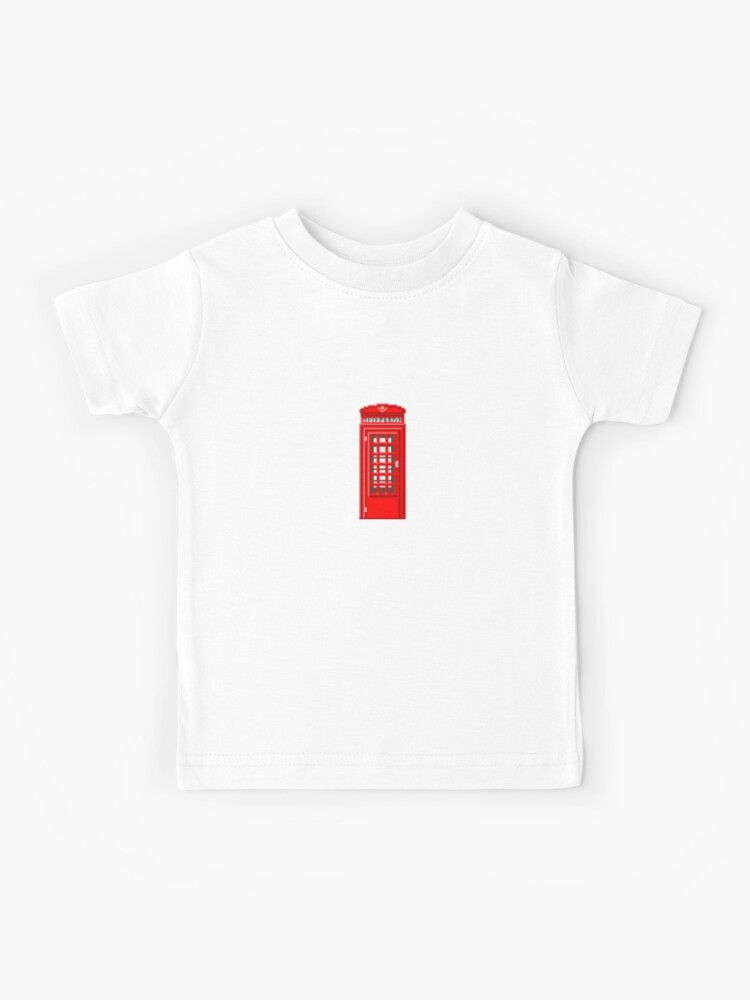This is an image of a small, short-sleeved, crew neck white t-shirt on a plain white background. Centrally positioned near the neckline is a detailed, upright red phone booth reminiscent of the iconic English-style design often associated with Doctor Who. The phone booth features a glass door with a grid pattern of three columns by five rows of panes, with matching grid work on the opposite side, allowing a glimpse through the booth. The door is adorned with a gold or yellow doorknob on the right and hinges on the left. Topping the phone booth is a domed area with white or yellow decorative elements just beneath its peak.